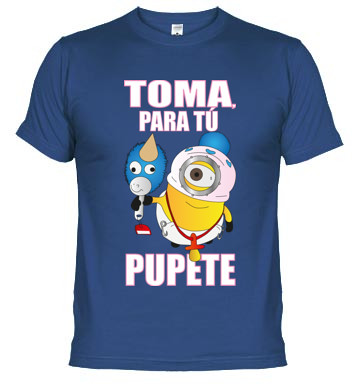The image features a dark blue T-shirt set against a plain white background. The T-shirt, styled with a typical U-line collar, has short sleeves stopping around the bicep area. The main graphic on the shirt showcases a character resembling a Minion from the "Minions" movie franchise. This character is depicted humorously, with a diaper over its head, allowing a hole for one eye to peek through, and another diaper worn conventionally. Around its neck hangs a red pacifier, and it clutches an item that appears to be a unicorn figurine. The image is accompanied by the text "Toma para tu pupete."